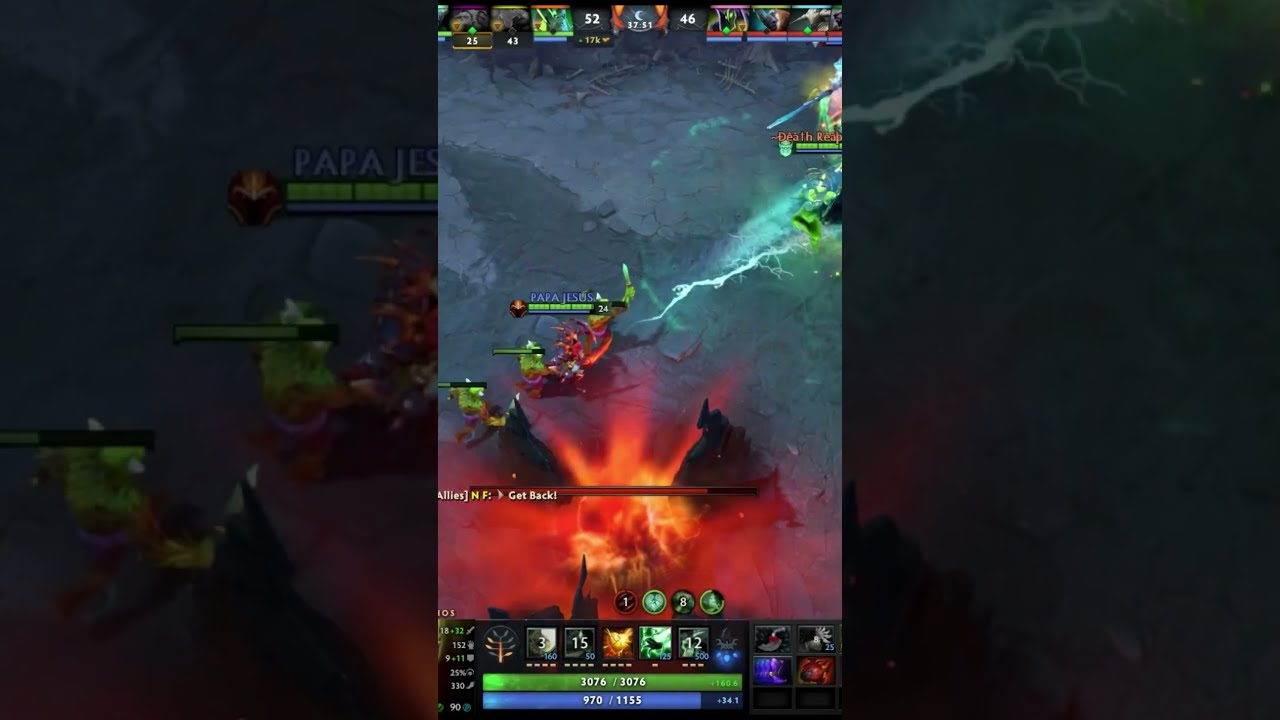This image is a detailed screenshot from a top-down mobile RPG game, set in a dark, dungeon-like environment characterized by a cracked, rocky terrain with a grayish-blue hue, suggesting a nighttime setting. The central part of the image features a heated battle between multiple small characters. Notably, there are three tall, green ogre-like warriors wielding swords, who seem to be attacking with lightning bolts. One of these ogres has been enlarged and placed on both the left and right sides of the full image for emphasis. On the receiving end of the attacks is a character named Death Reaper, discernible in bright green attire with blue hair. Death Reaper is accompanied by another warrior in red armor and possibly another figure in a white shirt. Health bars are visible above the characters, showing the current hit points, with one green line reading 3076 and another reading 970 out of 1155. At the bottom of the image, there is notable fiery activity with erupting lava from a volcano. Spell icons and additional game stats flank the battle scene, evoking a sense of a chaotic magical conflict with ongoing lightning and fire in the background.